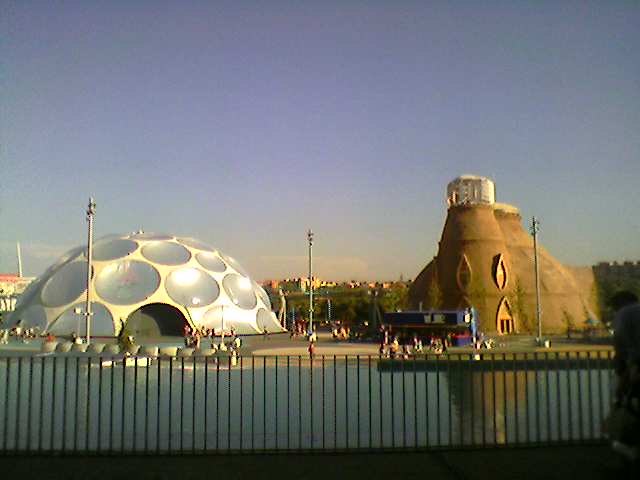The image depicts an outdoor scene at what appears to be an amusement park or tourist destination, possibly during the late afternoon as the sky exhibits hues of blue, pink, and a slight haze indicative of a setting sun. The foreground is dominated by a dark metal fence with small slats and a railing, behind which a calm body of water resides. Beyond the water, centrally located, a few people can be seen leisurely walking or standing near the shore.

Centered within the frame, behind the bodies of water and people, two striking buildings stand out. On the left, there is a large white dome adorned with silver circles and featuring a wide doorway, inviting visitors to enter. To the right, another unique structure appears, characterized by a brown dome with intricate windows and doors, fostering a fantasy-like allure.

The setting is enriched with various elements, including light poles, and a small blue building resembling a carnival game setup, elevating the amusement park atmosphere. The colors observed in the image—blue, light blue, gray, brown, orange, yellow, red, and silver—add vibrancy and life to this vivid depiction of a picturesque outdoor location.